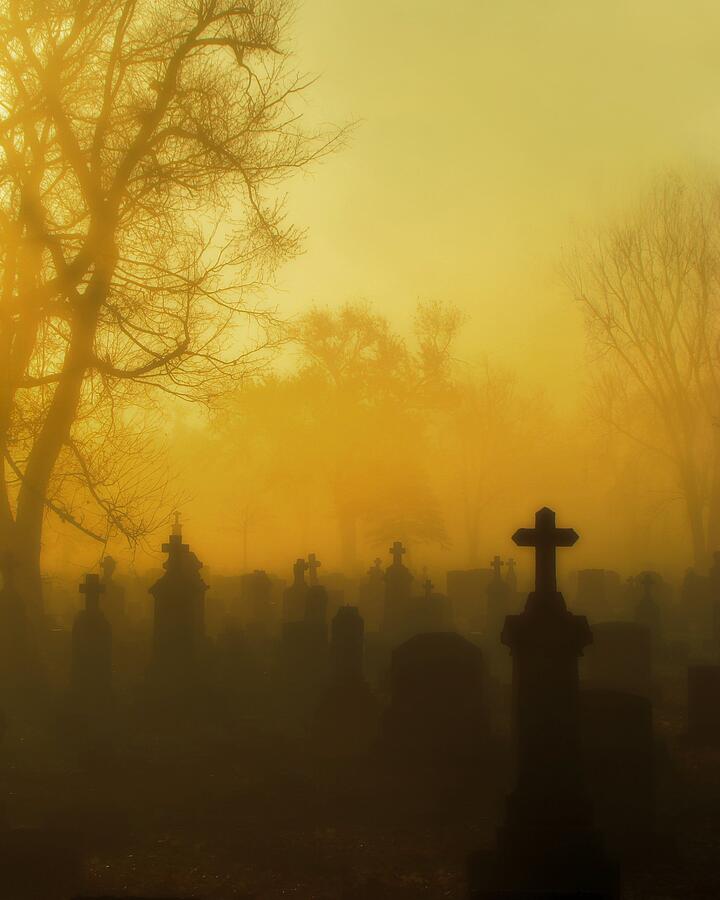In this haunting photograph of a graveyard, taken at either sunrise or sunset, the gravestones and barren trees form black silhouettes against a mesmerizing orange and yellow sky, giving the image a distinctly eerie and ambient feel. The sky bathes the scene in an amber hue, adding to the photograph's sepia, ghostly atmosphere. A prominent gravestone in the foreground, taller than the rest and topped with a stone cross, stands out in sharp relief. Surrounding it are numerous other tombstones of varying shapes and sizes, many also adorned with crosses, creating a somber and mysterious tableau. The trees flank the sides and stretch towards the middle background, their leafless branches adding to the stark, desolate mood of the scene. The photograph, characterized by its hazy, almost misty quality, offers little detail beyond the dark, shadowy forms of the gravestones and trees, enhancing its spooky, spectral impression.